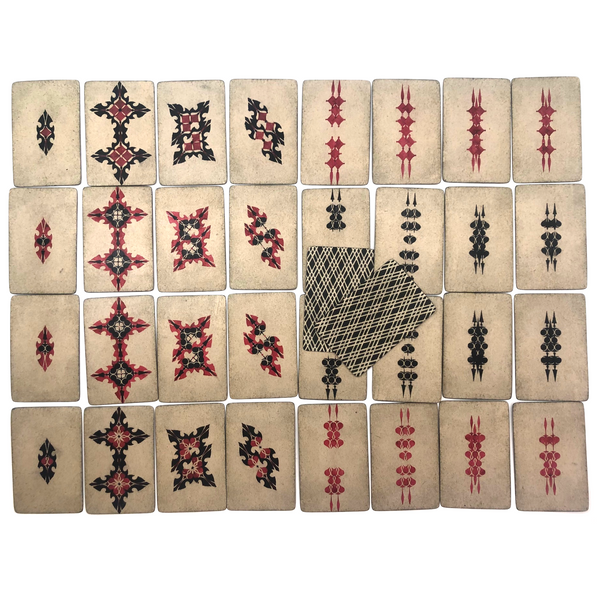The image depicts a grid of 32 playing cards arranged in a rectangular pattern of four rows and eight columns, all lying face down. These cards have a distinct Russian style and are primarily beige in color. Each card features traditional designs in dark blue and red at the center. The background of the image is plain white, creating a stark contrast with the cards, which appear to be old and faded. In the middle of the grid, two additional cards are placed face down in a criss-cross pattern, distinguished by their black and beige colors. The intricate designs on the cards include small diamond shapes, squares, and some spike-like and snowflake-shaped patches, hinting at their cultural richness and possible use in traditional or gambling settings.